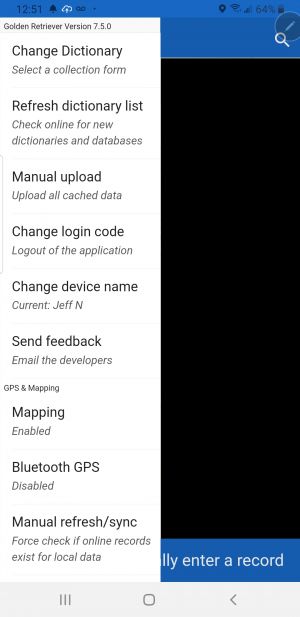The image showcases a user interface of a smartphone application with two distinct sections divided by their background colors. 

**Left Side of the Screen:**  
- **Background:** White  
- **Text:** Black  

Starting from the top: 
1. **Title:** "Golden Retriever Version 7.5.0"
2. **Options Listed Below the Title:**
   - Change
   - Dictionary
   - Select a collection form
   - Refresh dictionary list
   - Check online for new dictionaries and databases
   - Manual upload
   - Upload all cached data
   - Change login code
   - Logout of the application
   - Change device name (Current: Jeff)
   - Send feedback
   - Email the developers
   - GPS and mapping (Mapping enabled, Bluetooth GPS disabled)
   - Manual refresh or sync (First check if online records exist for local data)

**Bottom Left Corner:** 
- The options and descriptions continue with clear instructions and status updates related to GPS and data sync.

**Right Side of the Screen:**  
- **Background:** Black transitioning to blue at the bottom  
- **Text:** White

On this side: 
- **Top Right Corner:** There is a search bar or search icon with a white icon on a blue background.
- **Center Section:** Predominantly black background.
- **Bottom Section:** Blue background with white text saying "Manually enter a record."

Overall, the image presents a detailed and organized interface of the "Golden Retriever Version 7.5.0" app, providing numerous functionalities related to dictionaries, data management, and GPS mapping.